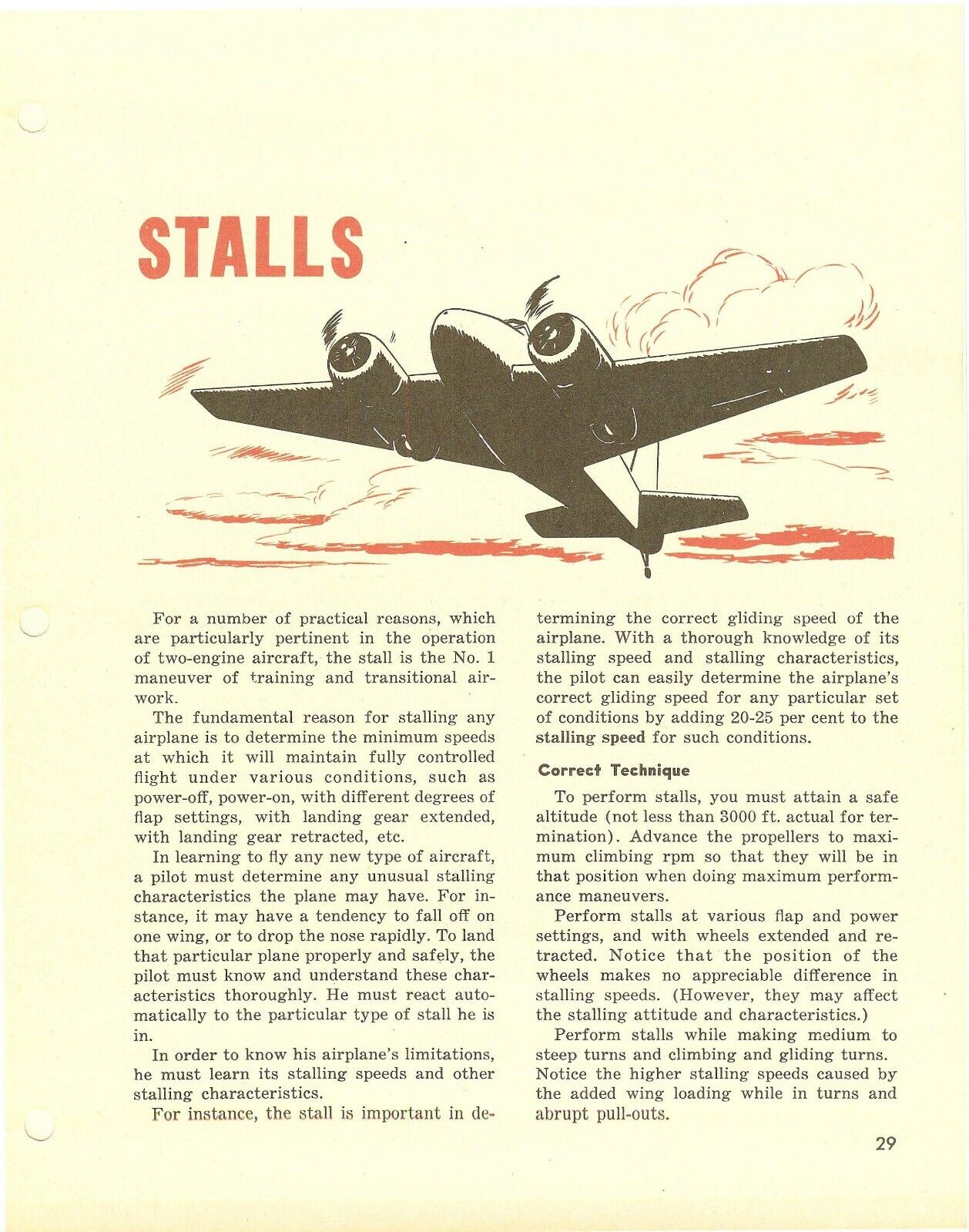The image depicts a yellowed page from a dated book with a focus on the aviation technique known as "stalls." A prominent black and white illustration of an airplane, primarily in shadow, is seen from a slightly upward angle with the reddish outlines of clouds in the backdrop, creating a dynamic perspective. The text is detailed and extensive, explaining that stalls are a critical maneuver for pilots, particularly in the operation of two-engine aircraft. The text elaborates on the functional reasoning behind performing stalls, such as determining the minimum speeds for maintaining fully controlled flight under various conditions, including different flap settings and landing gear positions. Key sections are highlighted in bold text, such as "stalling speed" and "correct technique," which offer step-by-step instructions for executing stalls safely. The page is punctured with hole marks on the left side, indicative of its place in a binder or an old manual, and is marked with the page number 29 at the bottom right. The content underscores the importance of understanding an aircraft's stalling characteristics and speeds to ensure safe landing and effective handling of the aircraft.